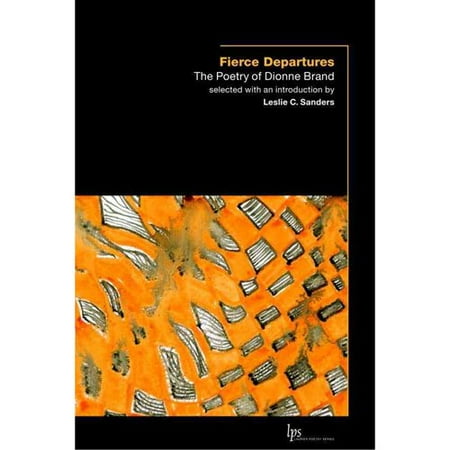This cover art for the book "Fierce Departures: The Poetry of Dionne Brand" features a predominantly black background. The title "Fierce Departures," printed in striking orange, is at the top, accompanied by a line shaped like an upside-down L above it. Below the title, in lighter text, is "The Poetry of Dionne Brand, selected with an introduction by Leslie C. Sanders," with Leslie C. Sanders' name slightly bolder. At the midpoint of the cover, there is a square image with an abstract theme: an orange background with black and white pieces, resembling floating paper fragments and childlike sketches of squares and lines. This visually intriguing abstract artwork adds depth and complexity to the cover. Toward the bottom of the cover, the initials "LPS" can be seen, followed by some illegible white text. This design sets a profound and artistic tone for Dionne Brand's collection of poetry, curated by Leslie C. Sanders.